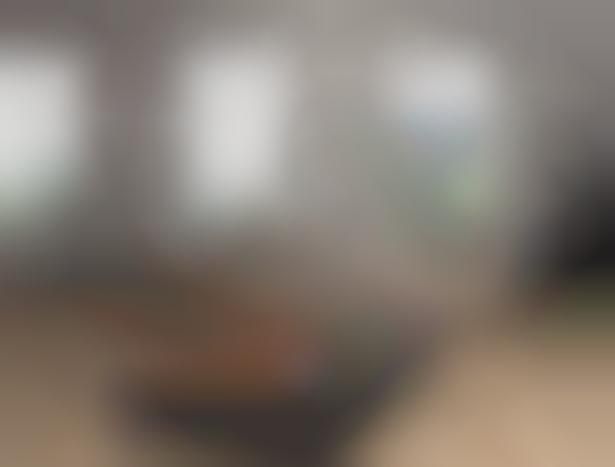The image is extremely out of focus and completely blurred, making it challenging to discern any distinct objects. The top portion of the image appears gray, transitioning to a whitish area towards the middle. Notably, there are three distinct white sections in the upper half, resembling the shapes of windows with light emanating from them. In the bottom half of the image, scattered blobs of beige are present predominantly on the left and right corners. Additionally, there's a mix of black, red, and green colors near the foreground, with the green possibly hinting at a body of water. Despite these color distinctions, the overall picture remains indeterminable due to the heavy blurriness.